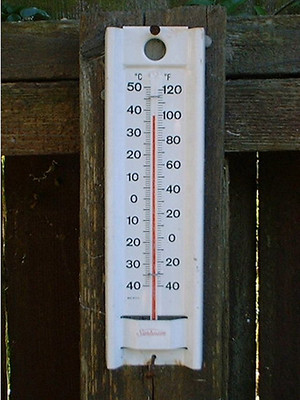This photograph showcases a long, white thermometer securely nailed to the main post of an aged, dark brown wooden fence. The fence, featuring visible wood grains and weathered panels, forms the rustic background of the image. The thermometer spans vertically from the top to the bottom of the frame, with a small circular cutout at its top for hanging. The temperature gauge, characterized by a slender tube with a red indicator line, displays temperatures in both Celsius and Fahrenheit. The Celsius scale on the left ranges from -40 to 50 degrees, while the Fahrenheit scale on the right spans from -40 to 120 degrees. At the bottom of the thermometer, there's a small indentation, adding a subtle design detail. The overall scene captures the contrast between the aged wood and the clean, utilitarian design of the thermometer.